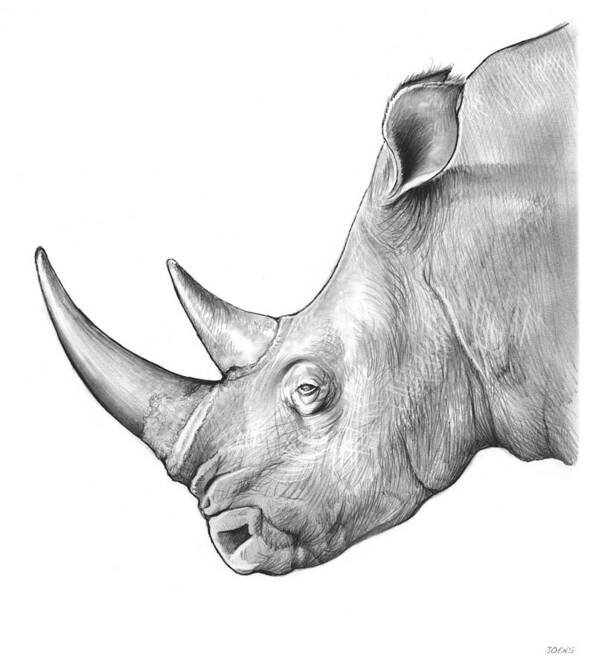This is an intricately detailed pencil drawing of a rhinoceros, showcasing its head in a striking side profile against a pristine white background. Rendered primarily in shades of gray, the rhinoceros's features are meticulously outlined, highlighting the pronounced snout and distinctive two horns— a larger one at the front and a smaller one behind it. The drawing also captures the animal’s textured skin with realistic shadows and wrinkles, skillfully depicted through precise pencil strokes. The rhinoceros’s tiny, almost closed left eye, surrounded by wrinkles, conveys a sense of depth and realism. Its ears, adorned with fine hairs sketched delicately around the edges, are set back on its head, as if the animal is attentive to sounds behind it. The light reflections on the horns and the face add a lifelike dimension to the image, making it an exceptionally visually appealing piece of art.